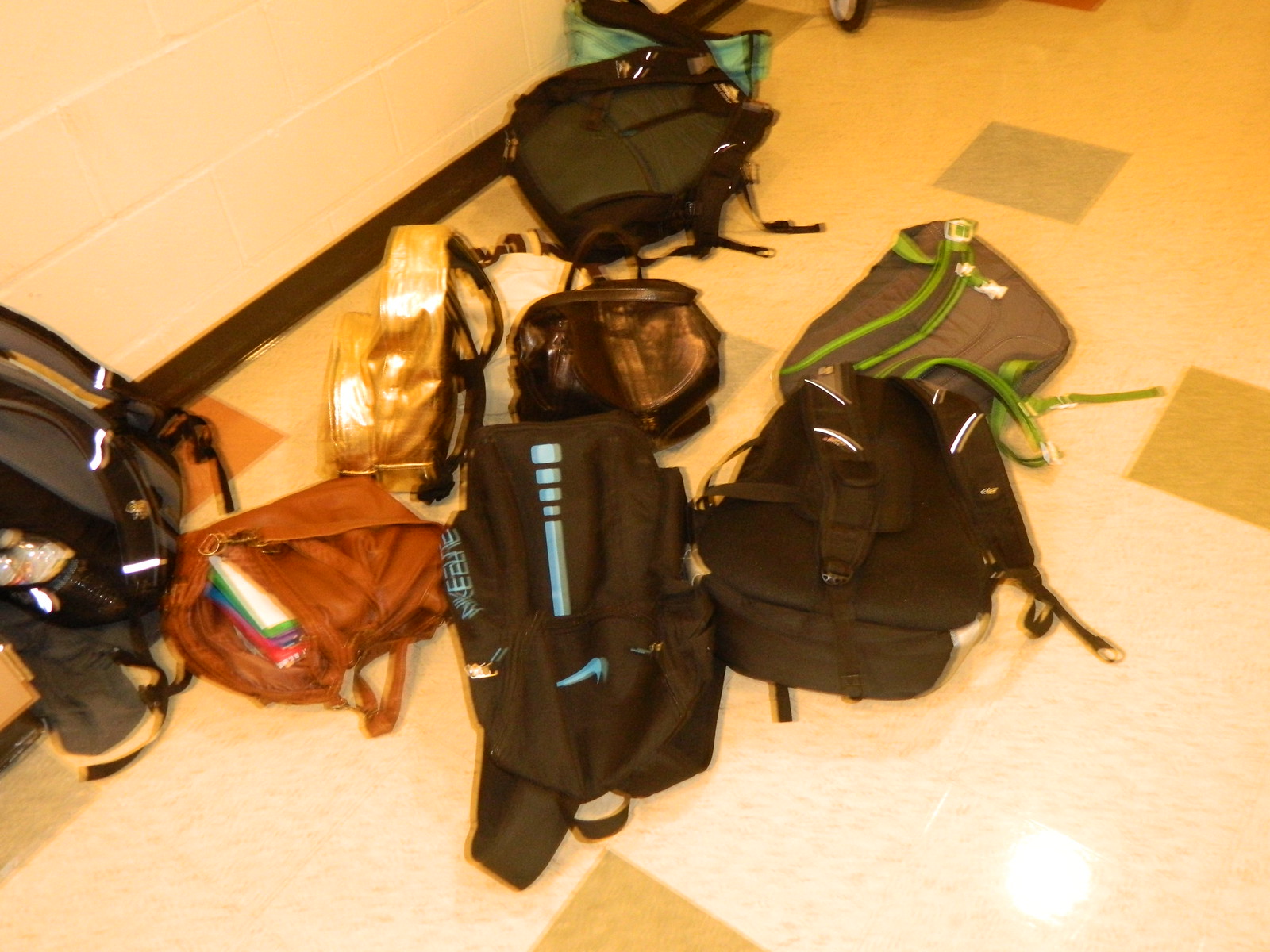This close-up, albeit slightly blurry photograph captures a cluttered hallway strewn with various school bags against a backdrop of white brick walls. The floor, predominantly formed of beige and white tiles, is interspersed with squares of gray, orange, and brown, creating a mosaic effect under the yellowish hue of fluorescent lights. The baseboards run along the hallway painted black, grounding the vibrant scene above. 

The focus shifts to an array of school bags, each with distinct features and colors, lying haphazardly on the floor. From left to right, a gray backpack is followed by a chocolate brown one, revealing books and folders within. Nearby, a shiny gold backpack catches the eye, contrasting with a smaller, two-toned chocolate and light brown bag. A gray bag with lime green accented straps sits adjacently, partnered with two predominantly black bags; one includes cyan accents, while the other showcases white stripes. Further back, a gray bag with black straps and another almost baby blue bag with black detailing round out the scene, all contributing to a snapshot of everyday school life, rich in casual disorder.